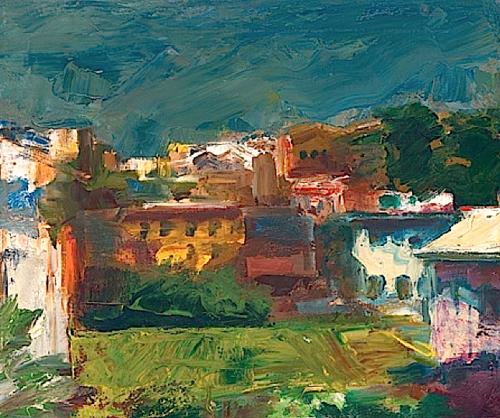The image is a watercolor painting, potentially using oils, depicting a vibrant, somewhat abstract town nestled amidst mountains or on a mountainside. The background features a swirled, textured dark blue sky. Centrally, a myriad of colorful buildings in hues of pink, blue, orange, red, yellow, and green overlap and blend into one another, creating a sense of dense urbanization or town life. These structures, ranging from small, hut-like homes to blocky, square buildings, give way to a scene that's bustling yet blurred. There are numerous dark windows visible across the buildings, suggesting occupancy and life within. To the right side, a brownish forest or cluster of trees adds a natural contrast. In the foreground, a green field with swirls of lighter green and yellow hues, along with bushes and various greenery, stretches out, adding texture and depth to the entire composition.